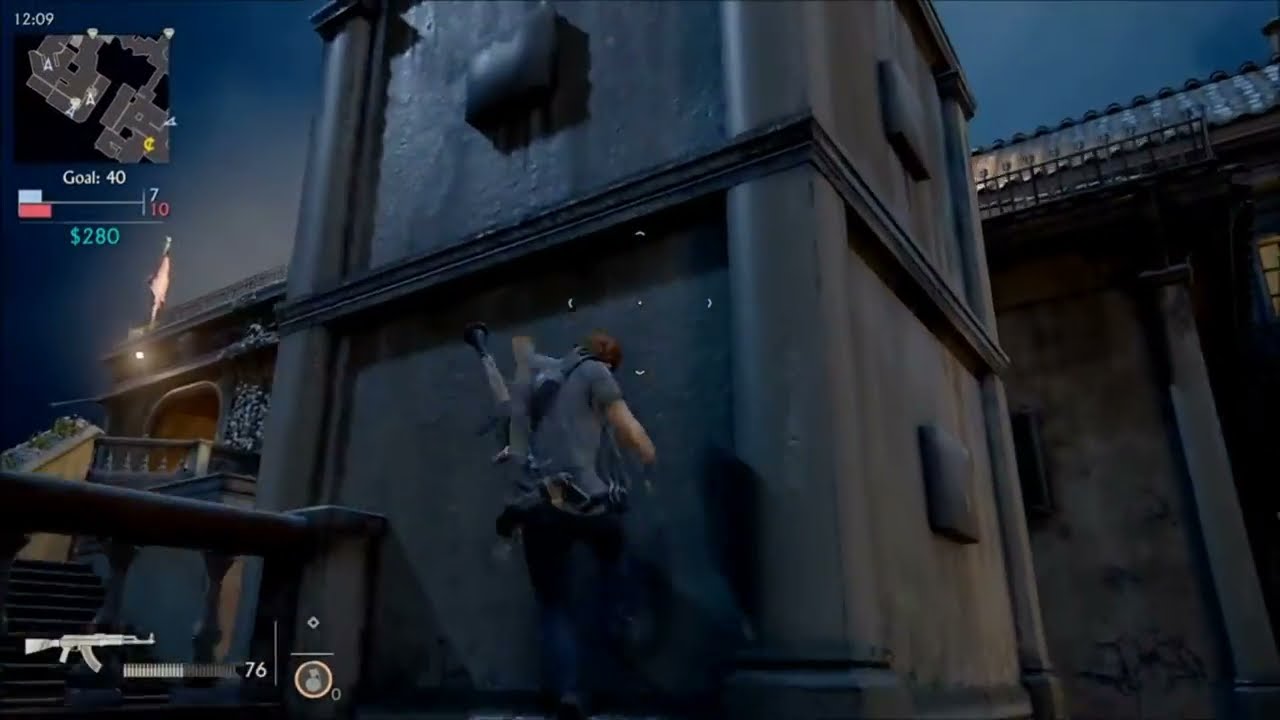This screenshot from a video game vividly captures an intense moment. The character, a male dressed in a gray shirt and dark pants, is seen scaling a two-story brown tower, gripping its sides with both hands. Above, in the darker, partly cloudy sky, indications of dawn or dusk set a dramatic backdrop. The top left corner of the screen displays a HUD with the time "12:09" and a map, suggesting the character's location and objective ("Goal: 40"). Below it, a white bar (quarter filled) and a red bar (slightly more than a quarter filled) can be seen, alongside "7" and "10," likely indicating health or other stats. The character's finances are also shown, with "$280" in green text. Positioned at the bottom left, an assault rifle icon, possibly an AK-47, is displayed, alongside an ammo bar halfway depleted, indicating "76 bullets remaining." To the right of the tower, a larger building with a fence-edged balcony and rustic tile roof reminiscent of Mediterranean architecture frames the scene. Stairs to the left lead into another structure, enhancing the complexity of the environment.